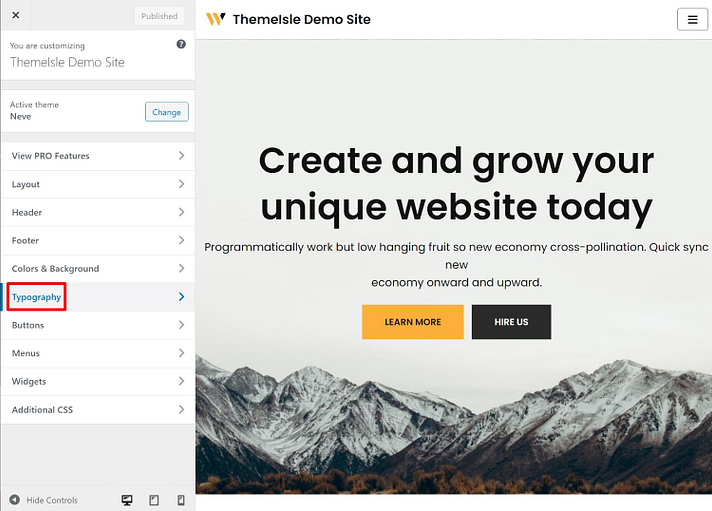This image is a screenshot depicting a demo site on a website creation platform similar to Shopify. At the top, the heading reads "Themso Demo Site," accompanied by a logo featuring a "W." On the left side of the screen, there is a dashboard with various options for editing the site, reminiscent of the Shopify interface. The dashboard includes a "Publish" button and indicates that the user is customizing the "Themso Demo Site" with the active theme labeled "Nev."

The customization options are presented as drop-down menus, including "View Pro Features," "Layout," "Header," "Footer," "Colors and Background," and "Typography." The "Typography" option is highlighted with a red box, signaling it is currently selected. Further down, additional options such as "Buttons," "Menus," "Widgets," and "Additional CSS" are accessible. At the bottom of the dashboard, there is an option labeled "Hide Controls."

The control panel also offers a preview feature with different viewpoints for desktop, iPad, and phone display modes. The demo site itself showcases an image of mountains under a gray sky, imparting a majestic feel. Overlaying this background, text prompts viewers to "Create and grow your unique website today," with actionable buttons labeled "Learn More" and "Hire Us," illustrating potential calls to action for the site.